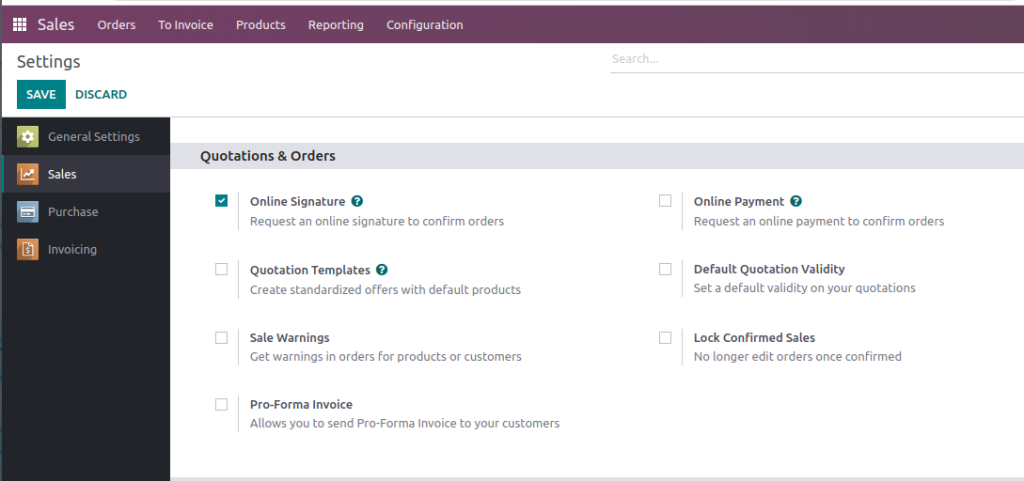**Detailed Description: Screenshot of Sales Software Interface**

The screenshot showcases an interface for sales software, characterized by a neat, modern layout with a combination of dark and light themes.

**Header Section:**
- **Top Header:** A prominent dark purple bar spans the top of the interface, displaying navigational options in white text, from left to right: Sales, Orders to Invoice, Products, Reporting, Configuration.
- **Secondary Header:** Below it is a white header with “Settings” written in black text. Positioned centrally within this header is an aqua-colored "Save" button. Adjacent to it in aqua text is the option to "Discard." On the top right of this header is a gray search underline with the text "Search" in gray placed above it.

**Left Sidebar:**
- The left section below the white header features a dark gray or black background divided into four categories, each marked by distinct backgrounds and icons:
  - **General Settings:** Highlighted by a green background with a white cog icon.
  - **Sales:** Identifiable by an orange background with a white chart icon.
  - **Purchase:** Showcased by a blue background featuring a white credit card icon.
  - **Invoicing:** Noted by an orange background with a white paper icon featuring a dollar sign.

**Main Content Area:**
- The main, right-side section of the page starts with a white background transitioning to a light gray header with dark gray text stating "Quotations and Orders."
- Below, the core content area is white, compartmentalized into seven sections, each prefixed by a checkbox and a description:
  1. **Online Signature:** It has an aqua checkmark; the description reads, "Request an Online Signature to Confirm Orders."
  2. **Quotation Templates:** No checkmark; described as "Create Standardized Offers with Default Products."
  3. **Sale Warnings:** No checkmark; description reads, "Get Warnings and Orders for Products or Customers."
  4. **Proforma Invoice:** No checkmark; it reads, "Allows you to send proforma invoice to your customers."
  5. **Online Payment:** Positioned on the right side, no checkmark; description reads, "Request an Online Payment to Confirm Orders."

This detailed interface layout effectively displays the key functional areas and options available within the sales software, organized for easy navigation and usability.